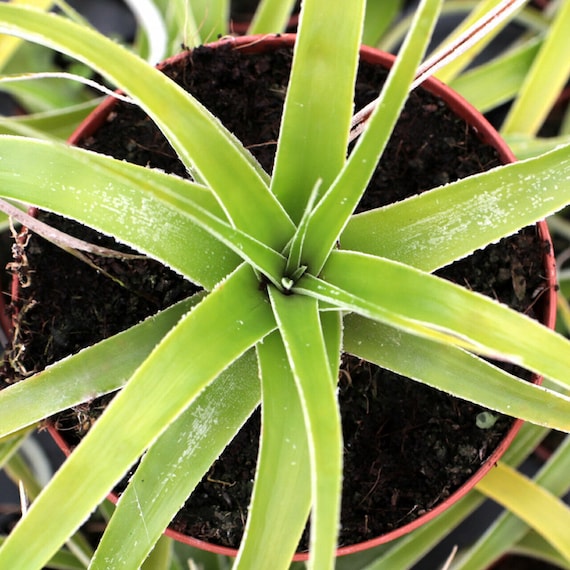This is an overhead, highly zoomed-in photograph of a succulent-style plant housed in a reddish-purple plastic planter. The plant sits in rich, dark potting soil, which is visible around the base. The focal point is the plant's long, thin, spear-shaped leaves that radiate from the center in multiple layers, totaling about 12 or 13 blades. The leaves are a vibrant green with thin, white stripes along the edges, giving a frost-like appearance. The tips of the leaves appear yellower compared to the deep green closer to the base. The image captures the emerging new leaves in the center, framed by the older, larger leaves extending outward. Surrounding this central plant are similar plants, adding depth and context to the scene.